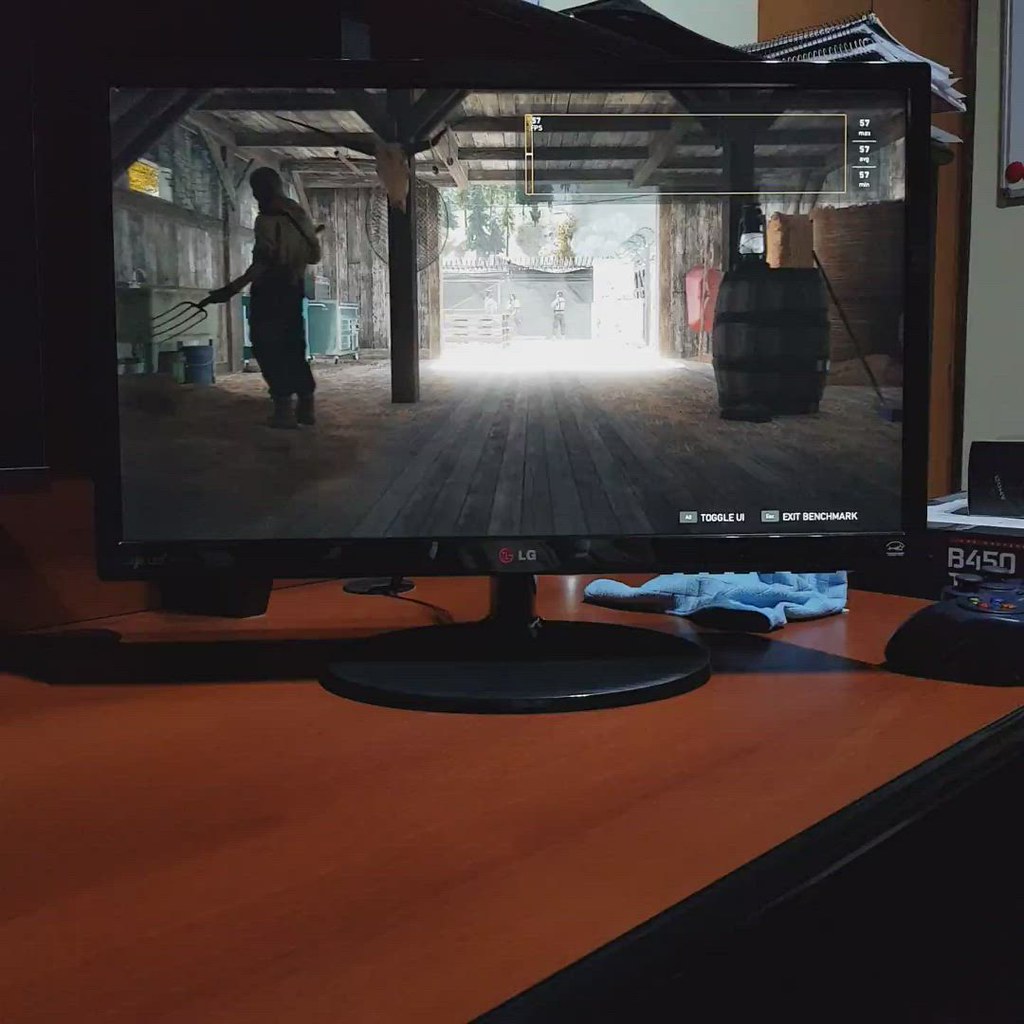The image depicts a detailed gaming setup. Centered on a brown desk, a black LG computer monitor features a circular base stand. Adjacent to the monitor, there is a game controller and a light blue towel positioned behind it. A few wires descend through a hole in the desk. On the left side of the desk, there is a box labeled "B450". 

The monitor displays an immersive video game scene set in a rustic barn or shed with lifelike graphics. The interior showcases light brown wooden walls and floors layered with hay. In the center, a character is seen from the back, holding a pitchfork. The character wears a beige shirt, long pants, and boots. Nearby, a window lets in daylight and a barrel sits atop a brown box. 

In the upper part of the screen, numeric data reads "57, 57, 57," accompanied by another figure and a yellow bar. Below this data, text reads "toggle LM" and "exit benchmark." 

Outside the main shed, across the scene, there is another tent-like structure with more characters. The daytime setting is further highlighted by a few visible trees and a red wheelbarrow leaning against the shed’s exterior wall.